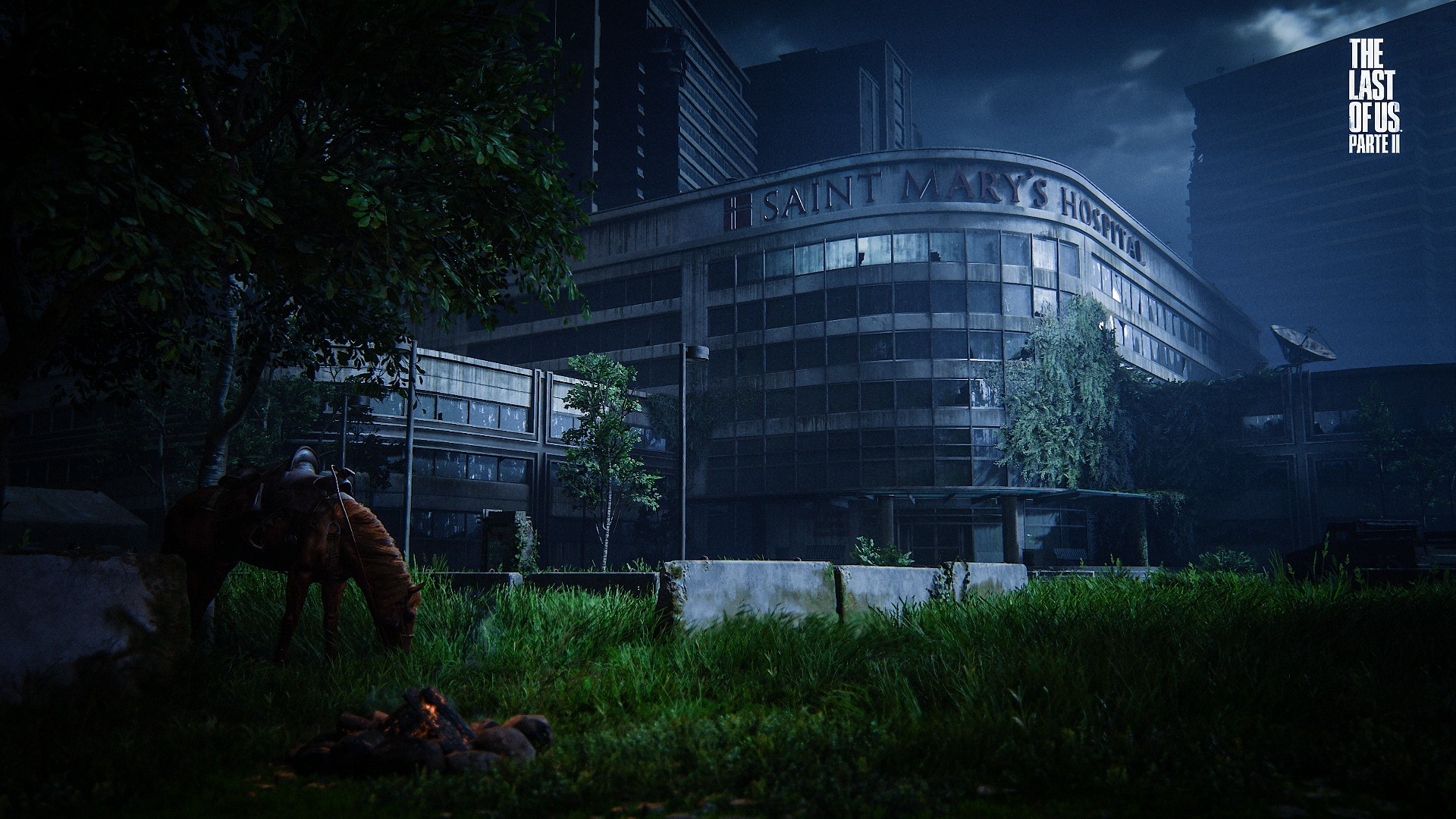The image is a detailed graphic from "The Last of Us Part 2," depicting a dystopian, post-apocalyptic cityscape at dusk. The centerpiece is a dilapidated St. Mary’s Hospital with darkened and broken glass windows, suggesting abandonment. The sky is stormy and heavy with clouds. Surrounding the hospital, much of the overgrowth includes green trees and overgrown grass, hinting at nature reclaiming the area. To the left of the scene, a brown horse with a saddle grazes near a small campfire, indicating a nearby human presence. Concrete bollards and stones creating a makeshift wall add to the rundown atmosphere. Against the backdrop of dark gray skyscrapers and a satellite dish, the bright green and brown hues of the horse and the grass starkly contrast, highlighting the desolate yet quietly vibrant life persisting in the foreground. The title "The Last of Us Part 2" is displayed in white text at the top right, enhancing the context of survival in a collapsed world.